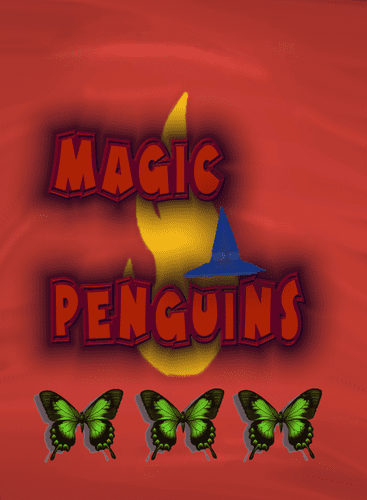The image features an artistically streaked background transitioning through different shades of red from left to right, creating a dynamic and fiery backdrop. Dominating the center are the words "Magic Penguins," written in a bold, comic-style font. "Magic" starts about a third down the page, while "Penguins" begins around 60% down, filling the space with impactful lettering.

Behind the text is a blue, almost witch-like or mage hat, positioned atop the letters "UIN" in "Penguins," extending upward until its tip nearly touches the "C" in "Magic." Enveloping this hat is a tall, narrow yellow flame that stretches from just below the "G" in "Magic" to the "I" and even from the "N" to the "C," giving the impression of a fiery aura.

Below the text and flame, aligned along the bottom at about 20% of the image, are three vibrant green butterflies with black-edged wings, reminiscent of monarch butterflies but without bodies. These butterflies have a high resolution, making them stand out sharply against the stylized background, as if they were pasted into the scene. The overall appearance suggests it could be a screenshot from a video game or a mobile app, characterized by its mix of detailed elements and stylized, clipart-like graphics.